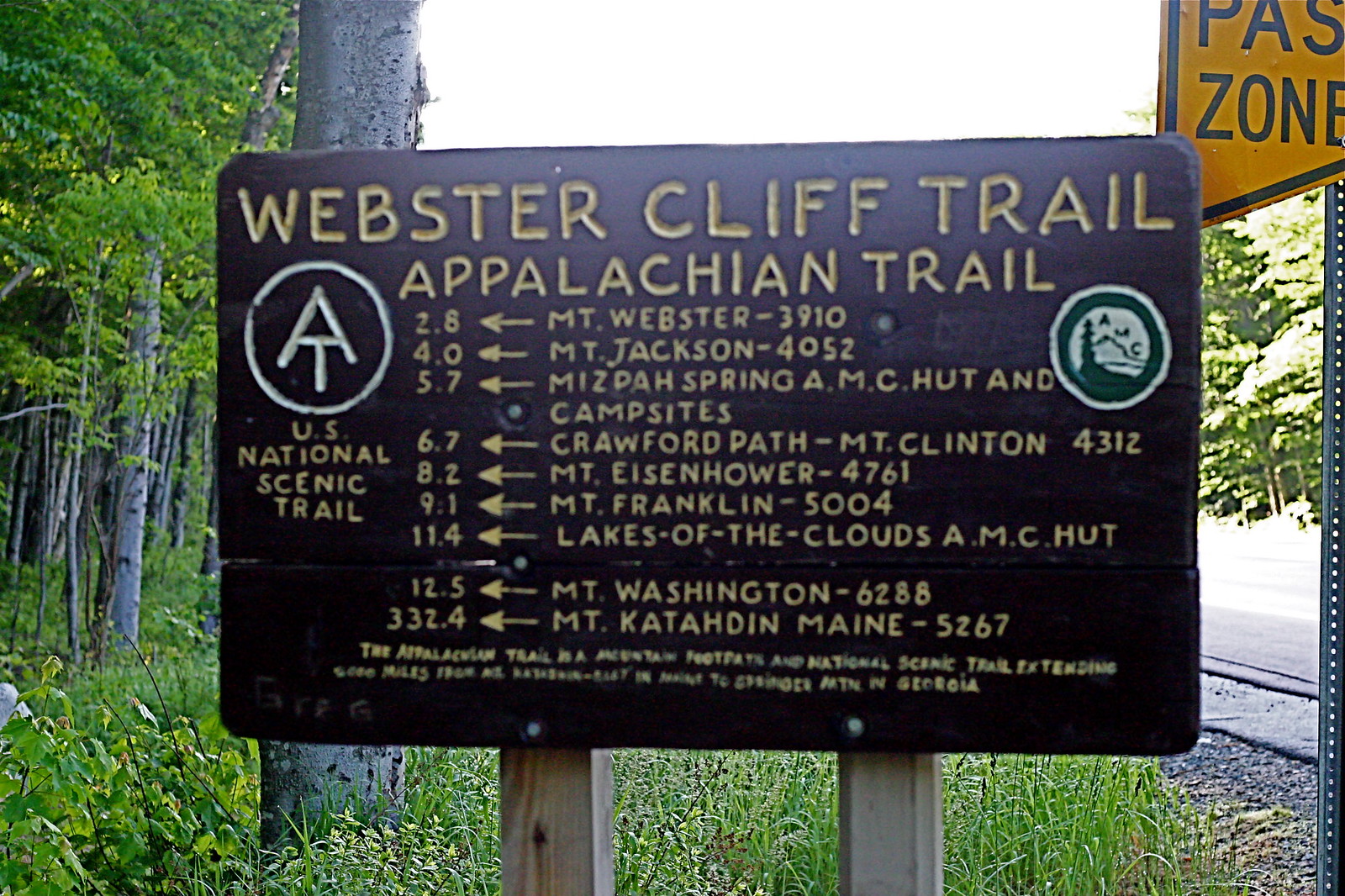This photograph captures a rectangular-shaped sign, prominently displayed as the central focal point. Taken outdoors in what appears to be a national or state park, the sign is supported by two wooden posts. The scene features a mix of natural and manmade elements: to the right, a roadway is discernible, indicated by a traffic yield sign and a yellow "pass zone" sign visible in the top right corner, partially cut off. To the left and behind the sign, a lush wooded area with birch trees extends into the background.

The sign itself has a rustic, weathered appearance, made of brown wood with bold yellow lettering. At the top, it reads "Webster Cliff Trail, Appalachian Trail, U.S. National Scenic Trail." Below this title, several locations are listed with corresponding distances and elevations, all directing hikers to the left. These include:

- 2.8 miles to Mount Webster, elevation 3,910 feet
- 4 miles to Mount Jackson, elevation 4,052 feet
- 5.7 miles to Mitzvah Spring AMC Hut and campsites
- 6.7 miles to Crawford Path, Mount Clinton, elevation 4,312 feet
- 8.2 miles to Mount Eisenhower, elevation 4,761 feet
- 9.1 miles to Mount Franklin, elevation 5,004 feet
- 11.4 miles to Lakes of the Clouds AMC Hut
- 12.5 miles to Mount Washington, elevation 6,288 feet
- 332.4 miles to Mount Katahdin, Maine, elevation 5,267 feet

Additional elements on the sign include a logo on the left, resembling a campground symbol, and a green and white "AMC" logo on the right. This detailed and informative sign is typical for guiding hikers along the Appalachian Trail, helping them navigate through various landmarks and scenic spots.